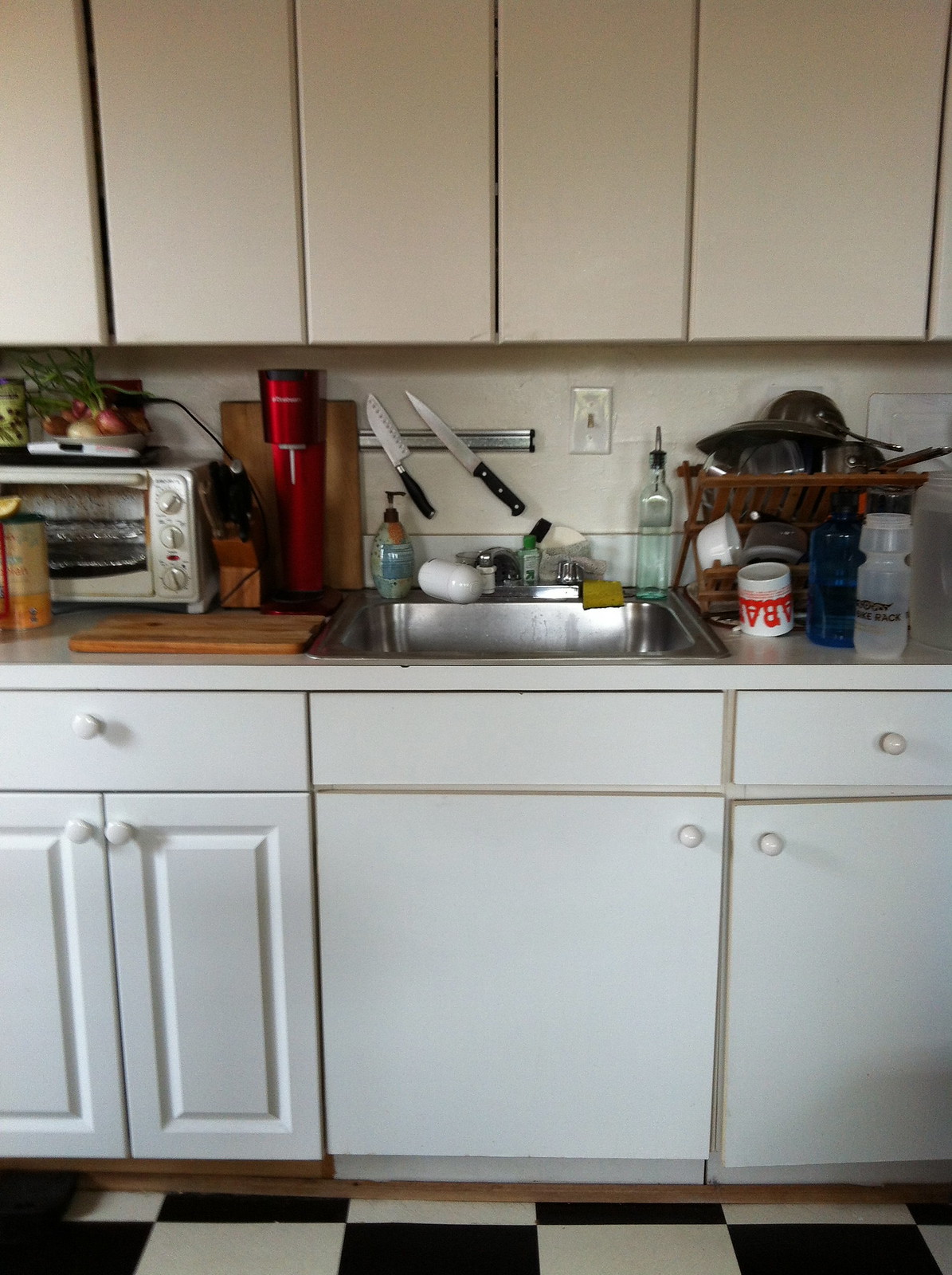The image showcases a meticulously detailed and charming kitchen interior. The floor features a classic black-and-white checkerboard tile pattern, lending a retro yet timeless feel to the space. The lower cupboards are painted white, adorned with matching white knobs, while the upper cupboards, also white, have a sleek appearance with no visible handles.

Central to the image is a metal sink, flanked by various kitchen essentials. Mounted on the wall behind the sink are a couple of knives, a handy and accessible storage solution. Nearby, a light switch is visible on the wall. Soap dispensers are positioned on both sides of the sink, indicating a well-organized and functional area.

To the right of the sink, a collection of items include a stack of dishes, a white coffee mug with red lettering, a clear plastic water bottle, and a brown dish rack overflowing with kitchenware. To the left of the sink, a vibrant red coffee maker adds a pop of color and is placed next to a leaning cutting board. Adjacent to these is either a completely metallic microwave or toaster oven, equipped with control knobs for setting temperatures. Atop this appliance, a variety of vegetables, possibly onions or radishes, are neatly arranged, adding a fresh touch to the kitchen scene. In front of the appliance, a brown can is conveniently placed.